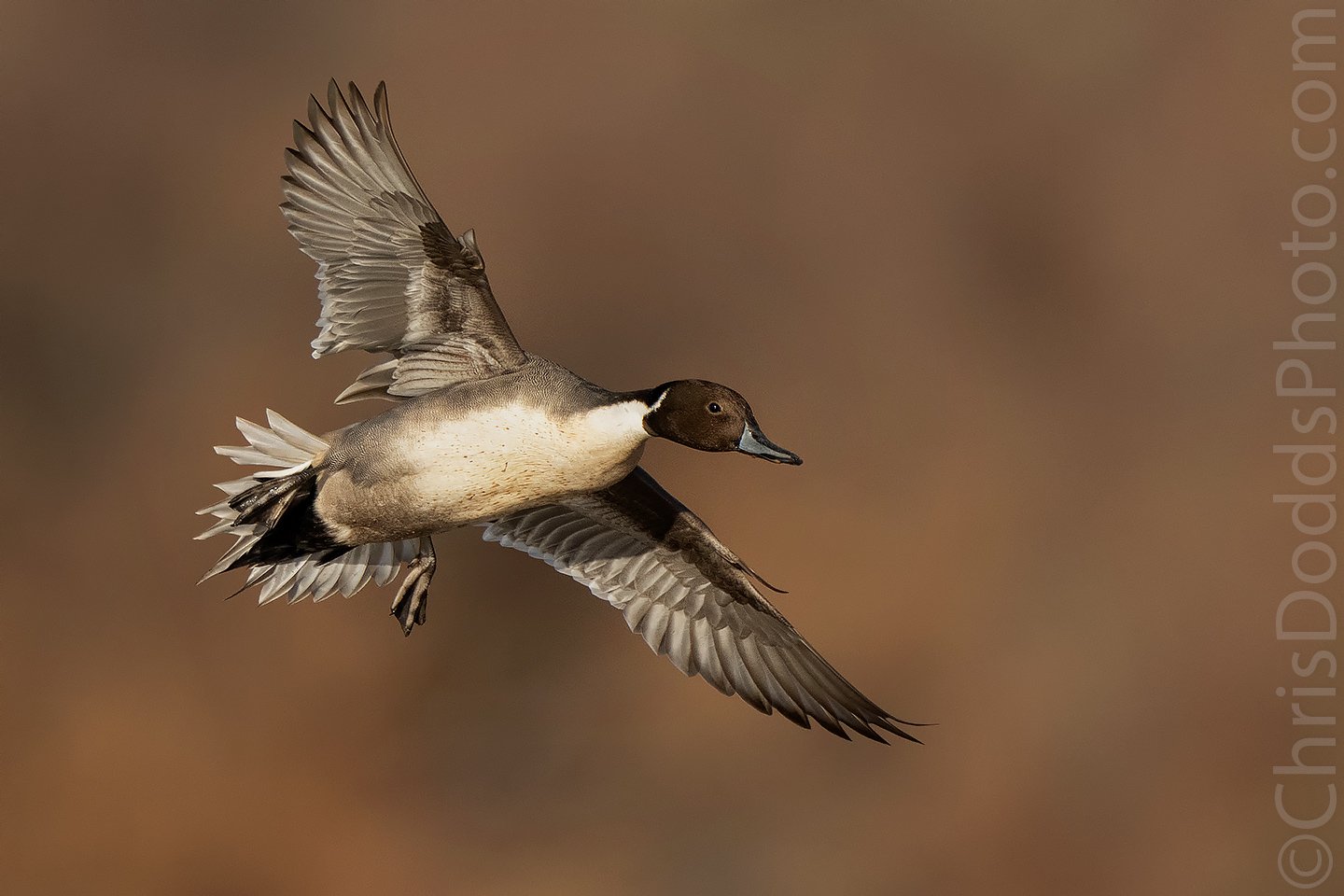This image showcases a close-up of a duck in mid-flight set against a blurred, brownish-tan background. The contrast between the sharp relief of the duck and the out-of-focus backdrop accentuates the intricate details of its widespread wings and tail feathers. The duck, positioned on the left side of the frame, is captured in a side profile facing right. It features a mix of tan, beige, and cream coloring with a light undersides and a downy texture. The duck's gray feet are faintly visible, complementing the creamy belly and distinct feather pattern that enables its graceful glide. The clear visibility of the duck's eyes and beak adds to the realism and vividness of the photograph. A watermark reading "© ChrisDoddsPhoto.com" runs vertically along the right side of the image, crediting the photographer.